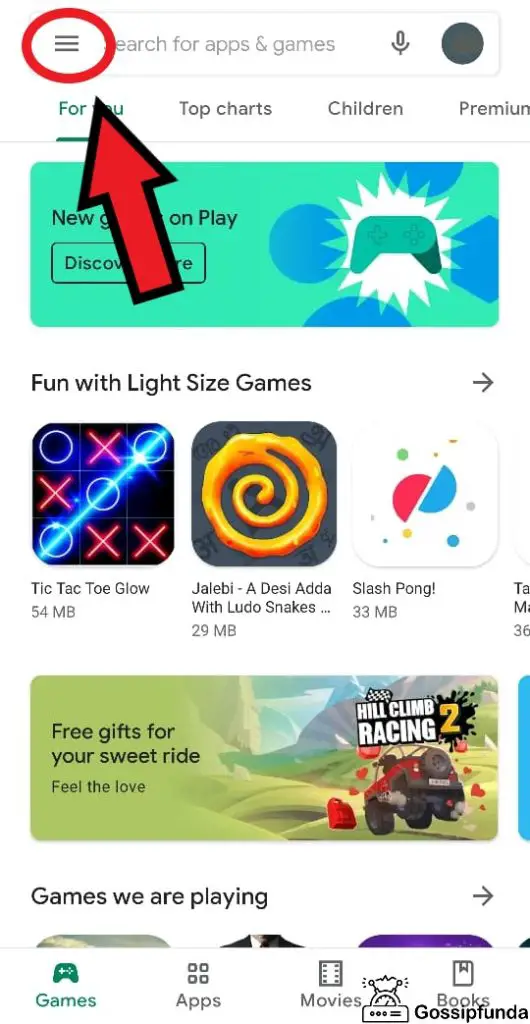A detailed screen capture of a smartphone displaying the Google Play Store app is used to illustrate specific steps in a tutorial. The focus is on the menu button, represented by three horizontal lines located adjacent to the search bar. This button is emphasized with a red circle and highlighted further with a large red arrow that features a black border, directing attention to the menu icon. The screen shows the default 'Games' section of the app, with categories like "New Games on Play," "Fun with Light-Size Games," "Games We Are Playing," and an advertisement for "Hill Climb Racing 2." A watermark labeled "Gossip Funda" is visibly present on the image, suggesting the source or creator of the content. The caption implies that the user is expected to access the menu for further actions, though the specific subsequent steps are not detailed within this image.